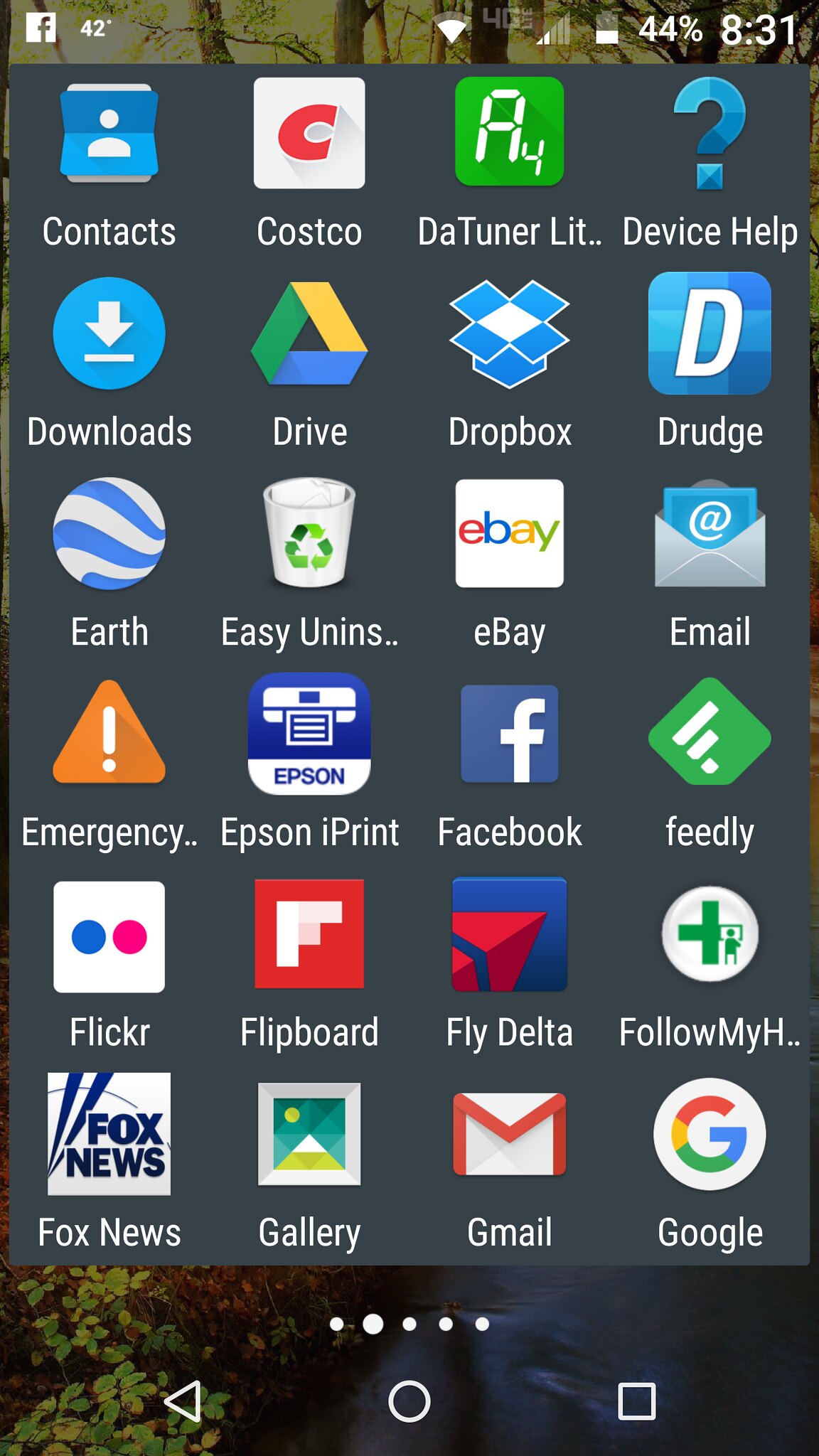This image captures a screenshot of a Samsung cell phone displaying its home screen. The phone's screen shows a 6x4 grid layout, comprising 24 app icons. The background wallpaper features a serene forest scene. 

At the top of the screen, the status bar provides useful information: the Facebook app is currently open, the temperature is displayed as 42 degrees, a strong Wi-Fi signal is indicated, the device is connected to a 4G network, the battery level is 44%, and the time is 8:31.

The app icons appear to be organized alphabetically. The top row includes "Contacts," "Costco," "Tuner," and "Device Help." The second row features "Downloads," "Drive," "Dropbox," and "Drudge." Continuing in alphabetical order, the third row displays "Earth," "Easy Uninstall," "eBay," and "Email." The fourth row lists "Emergency," "Epson iPrint," "Facebook," and "Feedly." Finally, the fifth row contains "Flickr," "Flipboard," "Fly Delta," and "Follow My Health," followed by "Fox News," "Gallery," "Gmail," and "Google."

Additionally, there are indicators at the bottom showing that this is the second page of the app menu, with five more pages accessible via swiping.